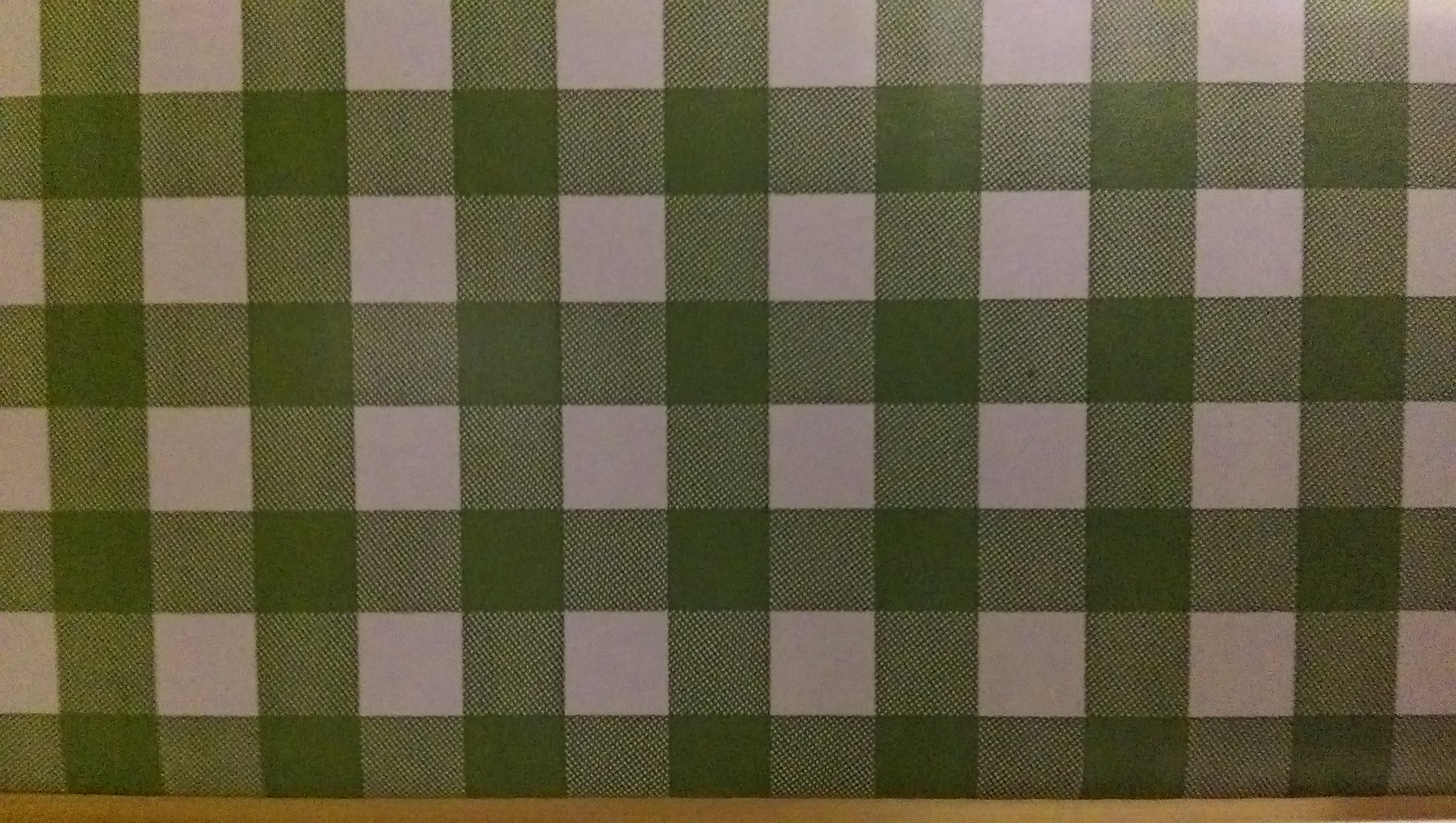This close-up photo showcases a piece of linen fabric featuring a green and white checkerboard pattern. The fabric forms a grid with four horizontal and seven vertical rows. The image, which is somewhat dimly lit and of amateur quality, reveals varying brightness, with the left side appearing lighter than the middle and right sides. At the bottom of the image, there's a thin, brown strip, possibly a cardboard backing or part of a frame. Additionally, the intersection of the green stripes appears darker, while the non-intersecting sections show some bleeding of the underlying tan fabric within the green areas. The fabric looks to be slightly unevenly lit and is zoomed in closely, highlighting its texture and pattern in significant detail.